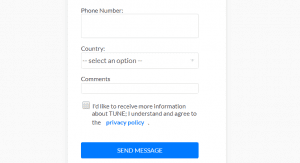The image shows a screenshot taken from a cell phone, displaying a form with a predominantly white background. At the very top of the form, there is a "Phone Number" label followed by a gray input box where a phone number can be typed. Directly below, there is a "Country" section, accompanied by an input box that reads "Select an option." Further down, the form features a "Comments" section, currently empty, but designed to accept user input.

Beneath the comments box, there is a gray checkbox labeled "I'd like to receive more information about TUNE" with the acronym TUNE in all capital letters. Following this statement, a phrase reads, "I understand and agree to the Privacy Policy," with "Privacy Policy" highlighted in blue, suggesting it is a clickable link for more information.

At the bottom of the form, there is a prominent blue button featuring white, capitalized text that reads "SEND MESSAGE." The form itself is set against a gray rectangular background, while all the form elements, including text and input fields, are contained within a vertically oriented white rectangle in the center of the image.